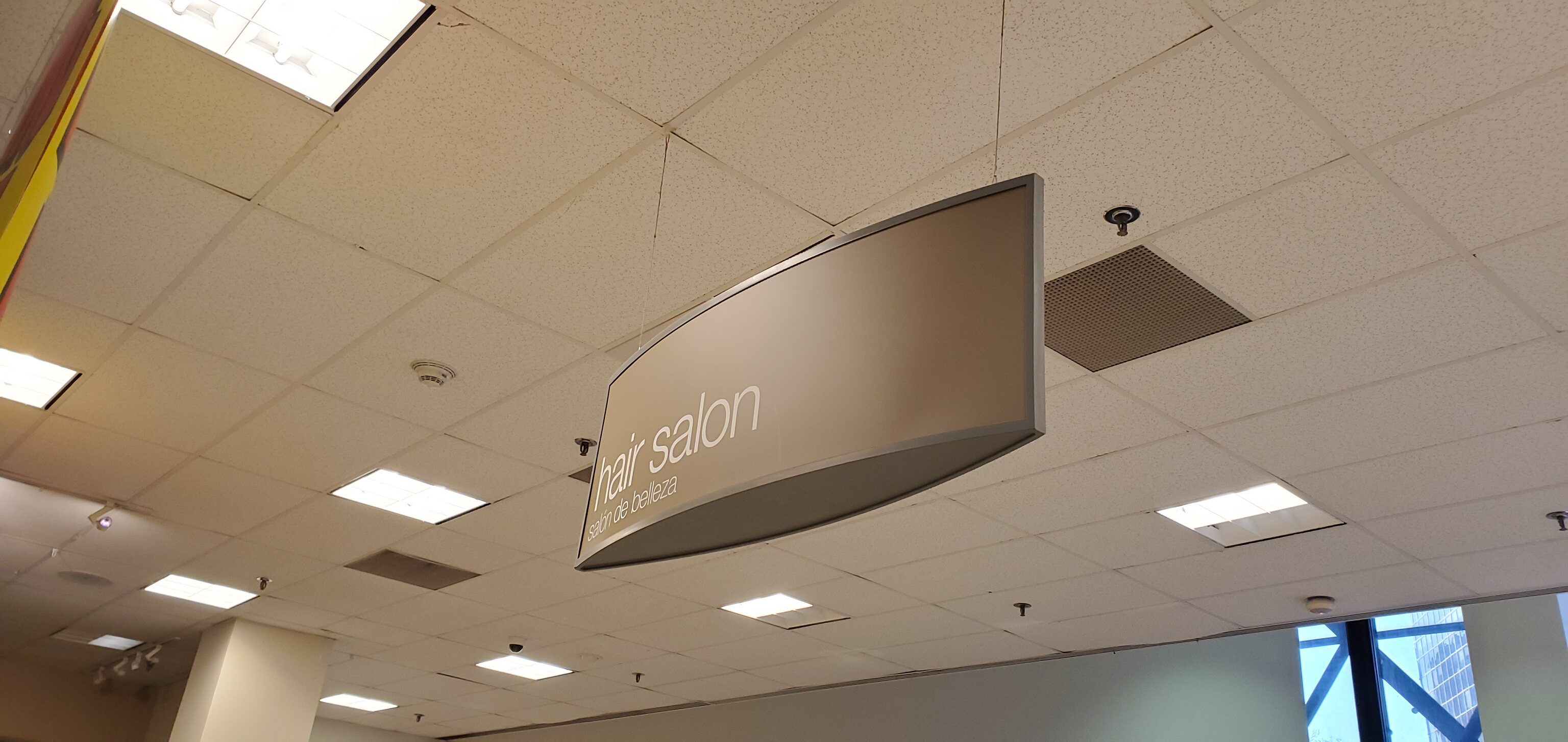A panoramic photograph captures an upward view of the interior ceiling of a building. The ceiling is adorned with square light fixtures that appear as bright white spots amidst the ceiling tiles. Featured prominently in the center of the frame is a curved, three-dimensional sign, gracefully bowing out on either side. The sign displays the text "Hair Salon" in the bottom left corner, with "Sabine de Beleza" written beneath it. In the bottom right corner of the image, a small window offers a glimpse of the outside world, revealing a pale blue sky.